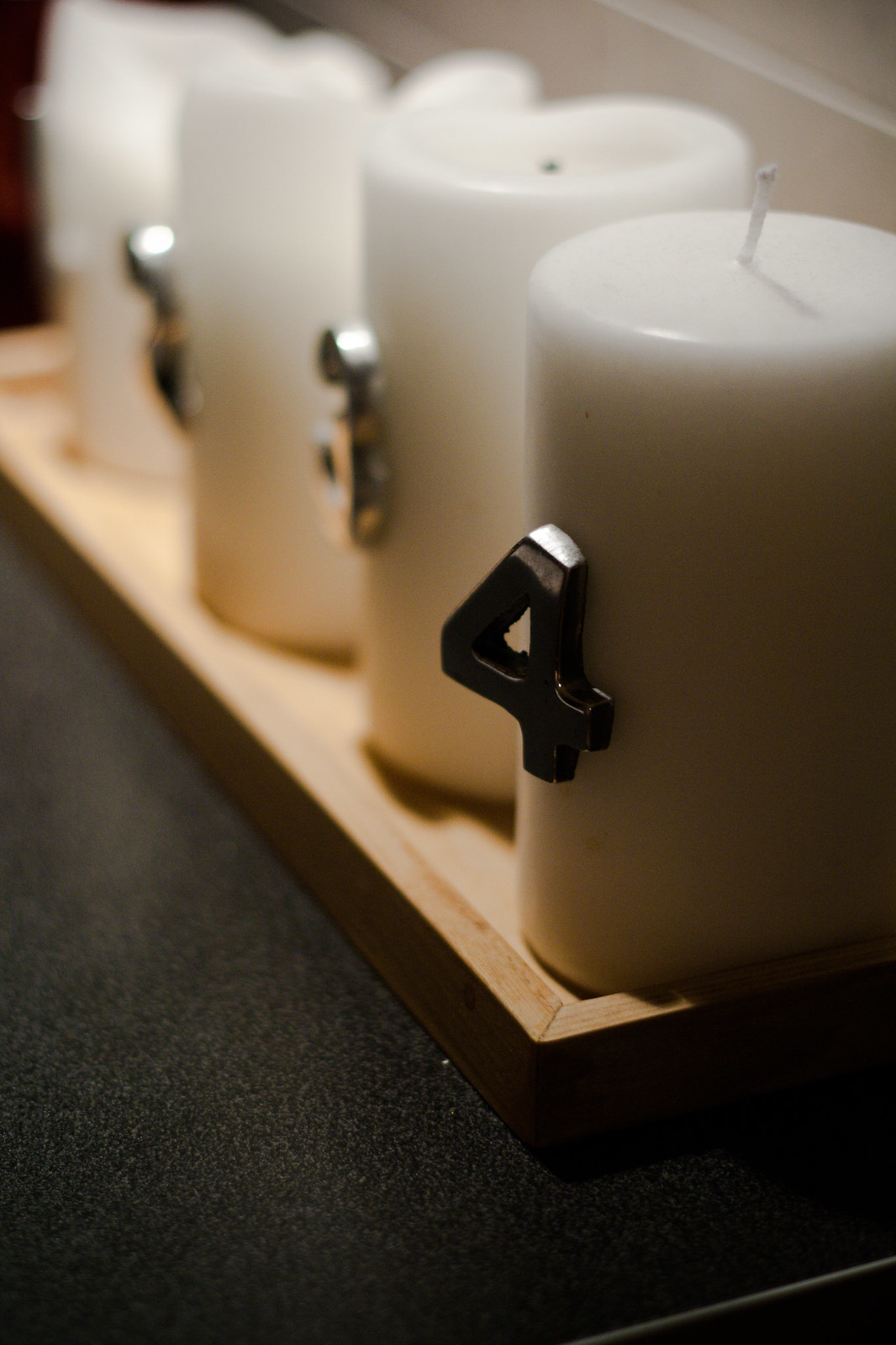The image depicts a close-up shot of four white pillar candles arranged in a straight line within a small rectangular wooden tray. The candles are numbered 1 through 4 with silver numerals affixed to their sides. The numbering and the focus of the image create a progressive effect, with the number 4 candle being the closest and most clearly in focus, while the other candles become increasingly blurred as they recede into the background. Behind the candles is a white wall, and the tray appears to be resting on a black surface, possibly a tabletop or cabinet. Each candle has been burned to varying degrees; the candle marked with number 1 is the most heavily burned and has the most wax melted, while the number 2 candle is slightly less burned, the number 3 candle has minimal burning, and the number 4 candle remains pristine and unlit. The arrangement and focus suggest an intentional gradation in the burning of the candles, likely for a decorative or symbolic purpose.